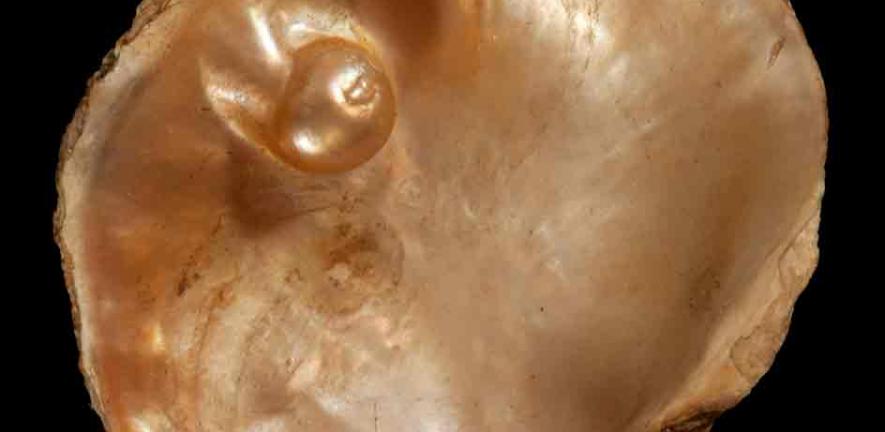This detailed close-up image captures the glossy, undulating interior of a medium to light brown, slightly metallic-looking shell, possibly from a clam or oyster, set against a stark black background. The object, which is oval-shaped, takes up most of the frame with the top and bottom quarters cut off, offering a view that focuses on the middle portion. Its smooth but wavy surface exhibits minor imperfections, including streaks, scratches, and chips. Notably, there are a couple of smaller sub-circles within the main form, one of which—located on the top left—resembles a pearl, enhancing the suggestion that this could be a seaside object. The lack of additional context or distinguishing features leaves some ambiguity, yet the shiny, undulating surface and the repeated mention of its shell-like appearance provide strong clues towards its identification.